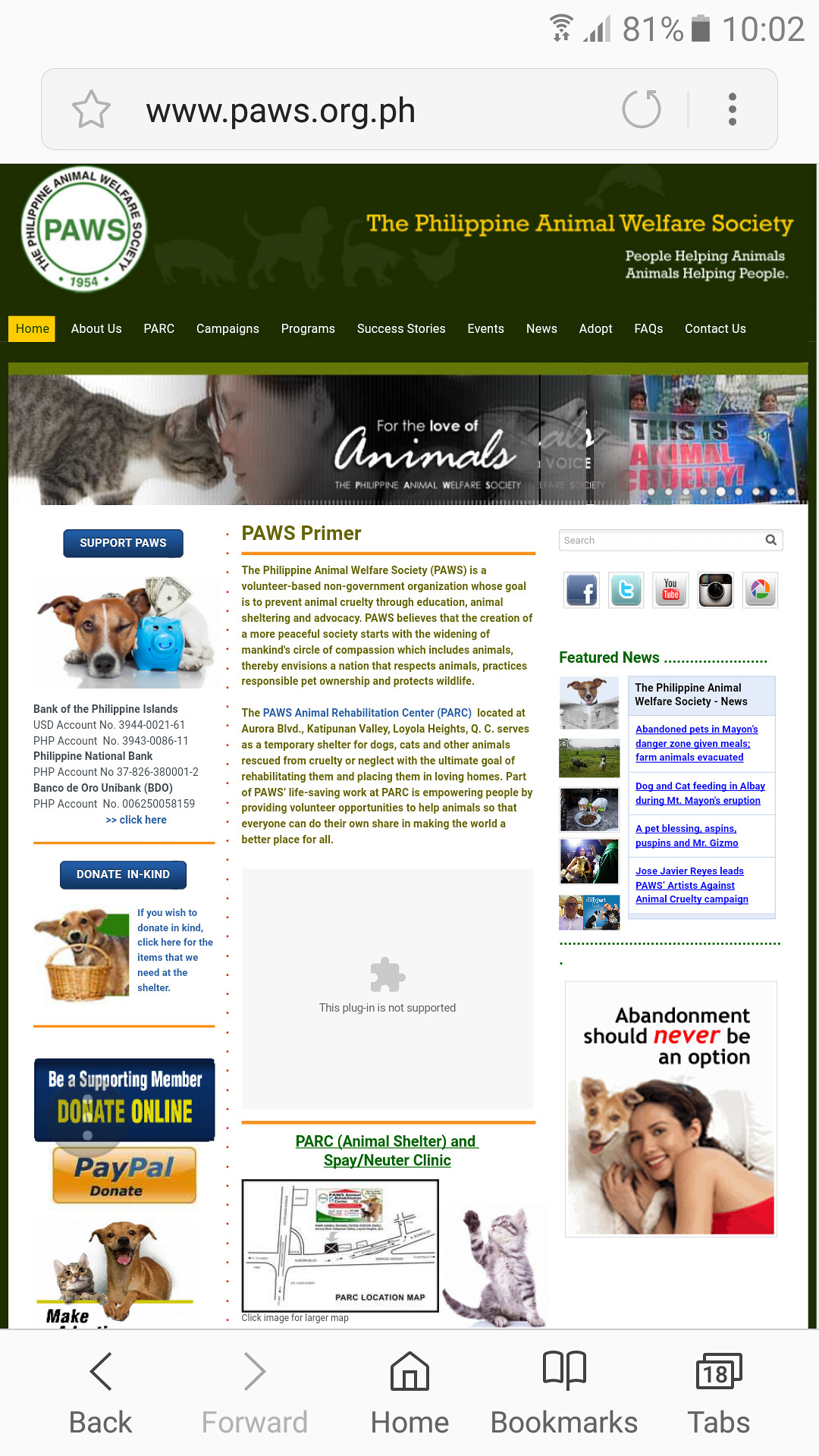This image is a screenshot of a mobile phone displaying the website for the Philippine Animal Welfare Society (PAWS) at www.paws.org.ph. At the top of the screen, the Wi-Fi emblem, signal bars, battery level at 81%, and the time displayed as 10:02 are visible. Beneath the browser address bar, which resembles Chrome, there is a green banner featuring the organization's name and slogan: "The Philippine Animal Welfare Society - People Helping Animals, Animals Helping People." The banner also includes lighter green silhouettes of various animals including a pig, dog, cat, chicken, and a jumping dolphin, along with the PAWS logo on the left side marked with "1954."

The website has a navigation menu listing links such as Home, About Us, PARC, Campaigns, Programs, Success Stories, Events, News, Adopt, FAQ, and Contact Us. The main content of the webpage is divided into multiple sections. Prominent among these are Feature News, PAWS Primer, Support PAWS, and Donate in Kind options, as well as PayPal donation links. The PAWS Primer section describes PAWS as a volunteer-based, non-governmental organization aimed at preventing animal cruelty through education, sheltering, and advocacy. It emphasizes the importance of compassion towards animals and outlines the mission of the PAWS Animal Rehabilitation Center (PARC) in Loyola Heights, QC, to rehabilitate and rehome rescued animals. Various images of adorable animals, such as pigs near piggy banks and a kitten waving, populate the white background of the page. At the bottom of the screen, navigation buttons for back, forward, home, bookmarks, and tabs are also visible.